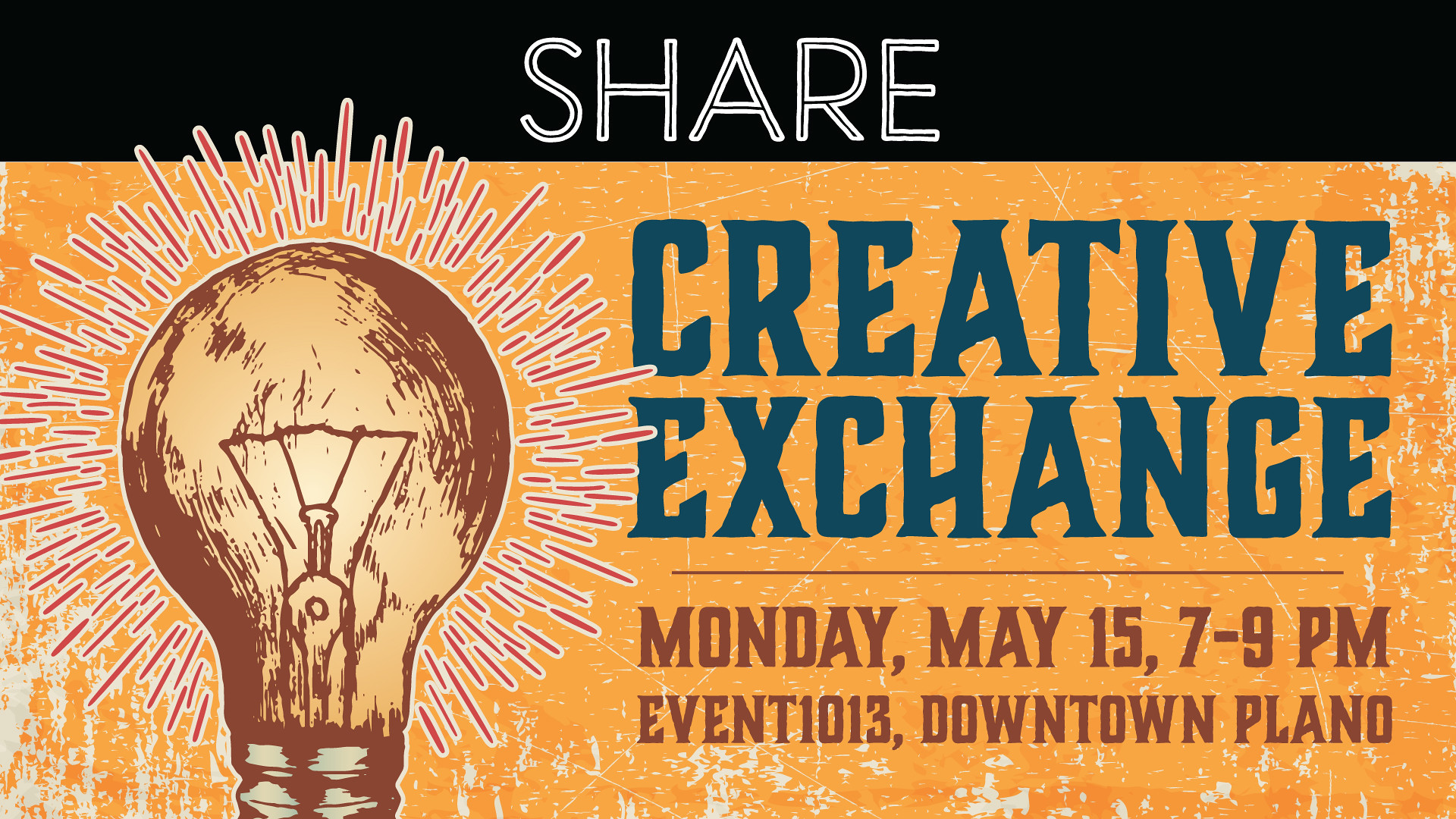The image depicts a business card-like design set against an orange background with a weathered, spray-painted texture featuring patches of white, giving it a scraped and aged appearance. At the top, a black strip runs horizontally across the card, with the word "SHARE" prominently displayed in bold, white, all-capital letters with a slight black outline. Below this, the bottom portion of the card is a textured yellow, similar to being sponged on.

On the left side of the card, there is an illustration of an Edison bulb, colored in shades of brown and gold, clearly showing the filament inside and the silver screw base at the bottom. The bulb emits rays of light depicted in a pinkish-gray color, giving a sense of movement and energy.

To the right of the bulb, the text "CREATIVE EXCHANGE" is displayed in blue, all capital letters, followed by a brown line underneath. Below this line, brown, all-capitalized text reads "MONDAY, MAY 15, 7-9 P.M." Continuing further down in smaller, all-capital letters, it states "EVENT 10 13, DOWNTOWN PLANO". This card appears to promote an event aimed at gathering like-minded individuals to share ideas and creativity.